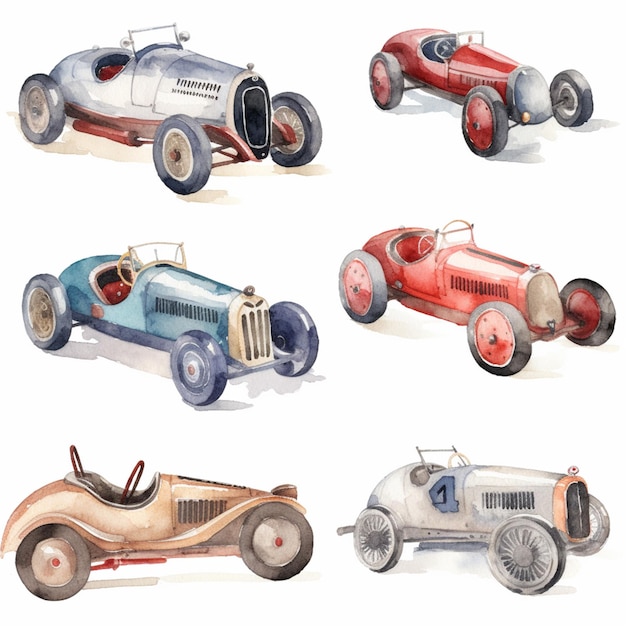The image showcases a series of six vintage racing cars, meticulously hand-drawn and colored using watercolor paints. The cars are arranged in three horizontal rows of two. Each car features a long, rectangular body with a distinctive curved back behind the driver's seat and an elongated front with a flat yet curvy grill. All vehicles boast four large wheels, either fully exposed or adorned with curvy fender flares.

In the top row, the car on the left is silver with a contrasting red bottom, while its neighbor on the right sports a red body and a silver front end. The middle row displays a blue car on the left, enhanced with a darker blue bottom, and a red car on the right, deepened further by a redder lower half. The bottom row holds an all-gold car in the left corner, with an all-silver one on the right, notably marked by a blue number one on its side.

Each car is uniformly designed as an open-top, single-cockpit vehicle, featuring a minimalistic small clear glass windshield in the front. The wheels match the body paint color, reinforcing their unique, unified aesthetic. The background of the image is stark white, drawing attention to the vivid and diverse hues of these nostalgically styled race cars.